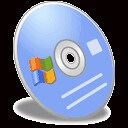In the center of the image, a digitally created depiction of an old Microsoft Windows CD dominates the scene. The disk, primarily light blue, features a gray edge and a black ring around the center point. The iconic Windows logo is present on the left section of the blue disk, displaying the familiar red-orange, green, blue, and yellow squares in a wavy pattern. Adjacent to this, on the right, is a plain white square. Two horizontal white lines, of equal length, run across the bottom portion of the disk. Below the CD, a circular gray base with a white ring creates a 3D effect, giving the illusion that the disk is propped up and casting a shadow. The entire composition is set against a stark black background. The image, distinctly cartoonish and reminiscent of the late 90s or early 2000s, expertly captures the nostalgic essence of older Windows software packaging.